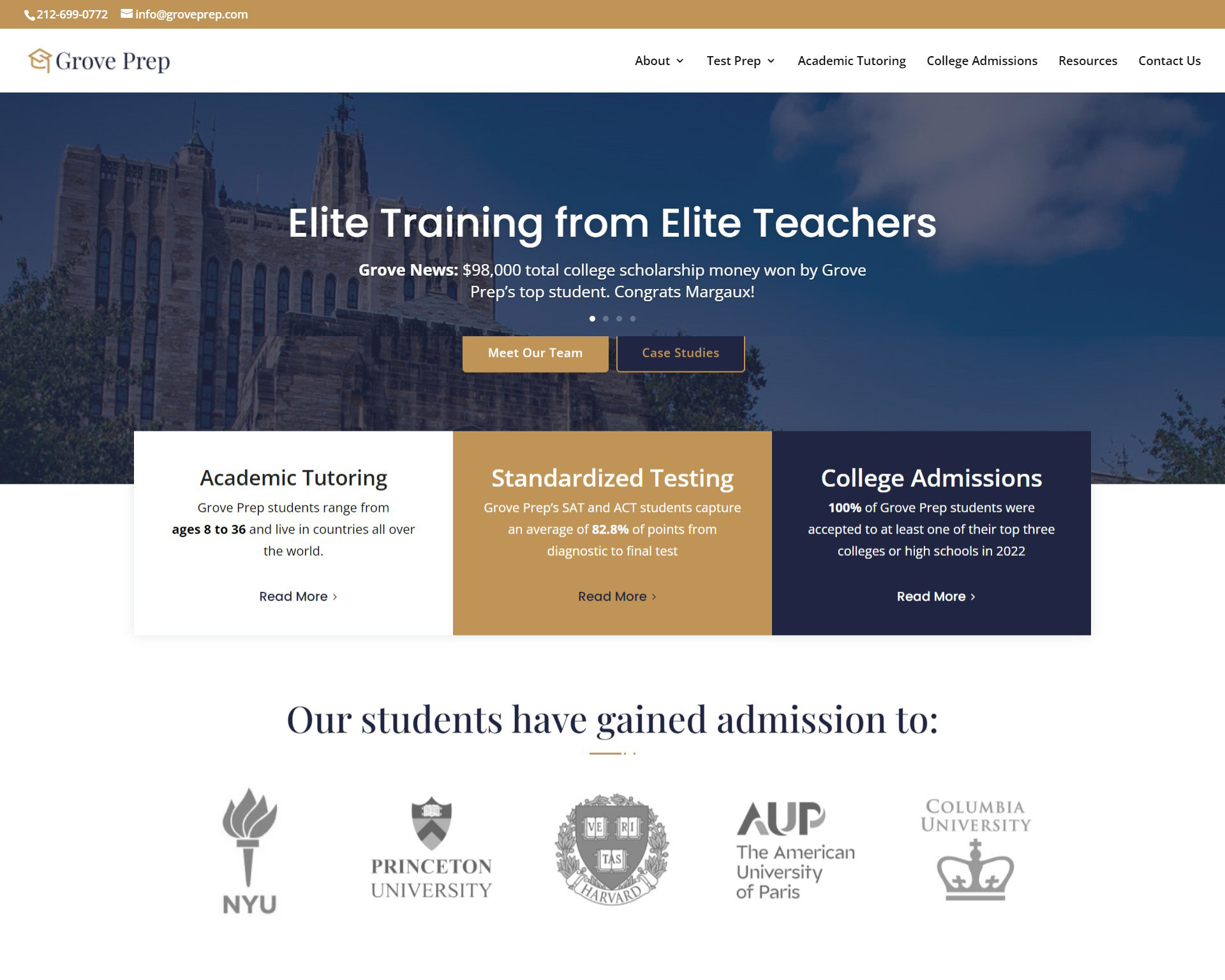This image is a detailed screenshot of a school website for Grove Prep. At the top is a gold-colored bar extending from the upper left to the upper right, displaying the school's phone number and email address. Below this bar is the school's name, "Grove Prep," accompanied by a minimalist line art logo resembling a graduation cap.

On the right-hand side of the screen, there are several navigational tabs: "About" and "Test Prep" have dropdown menus, while "Academic Tutoring," "College Admissions," "Resources," and "Contact Us" are clickable links. 

Beneath these tabs is a photograph of the school, which resembles an old castle, adding a historic and prestigious touch. Overlaid on the image is text that reads, "Elite Training from Elite Teachers." Below it, a news ticker states, "Grove News: $98,000 total college scholarship money won by Grove Prep's top student, congrats Margo." There are four small dots indicating additional news blurbs that users can click through to read more.

Two prominent buttons are centered beneath this section: one gold button labeled "Meet Our Team" and a dark navy button labeled "Case Studies." 

Further down, three distinct informational boxes are displayed in different colors: "Academic Tutoring" in white, "Standardized Testing" in gold, and "College Admissions" in navy. The "Academic Tutoring" section notes that Grove Prep students range from ages 8 to 36 and come from various countries worldwide. It highlights Grove Prep's impressive statistics: their SAT and ACT students capture an average of 82.8% of points from diagnostic to final test, and 100% of their students were accepted to at least one of their top three college or high school choices in 2022.

Additionally, the site proudly lists notable universities where their students have gained admission, including NYU, Princeton University, Harvard, the American University of Paris, and Columbia University, with the corresponding logos of these institutions displayed below.